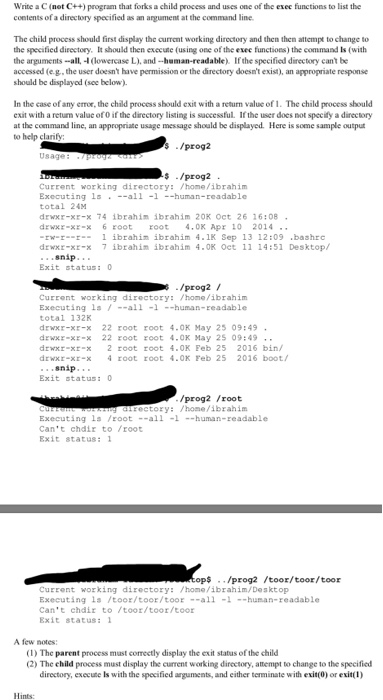This image showcases a desktop screenshot that appears to display a PDF document, though the specific browser or operating system is undetermined. The document contains extensive text related to writing a C (not C++) program involving creating a child process via forking and executing a directory listing command using an exec function. Some sections of the document have been redacted.

The main task illustrated in the document involves writing a C program where the child process must:
1. Display the current working directory.
2. Attempt to change to a directory specified by a command line argument.
3. Execute the `ls` command with the arguments `--all -l --human-readable` to list directory contents.

If the specified directory cannot be accessed, the child process should provide an error message and exit with a return value of 1. Successful directory listing should result in an exit value of 0. The document emphasizes the importance of displaying a usage message if no directory is specified and correctly communicating the exit status of the child process through the parent process. 

Examples of output provided include displaying the current working directory (`/home/Ibrahim`) and executing the `ls` command with the appropriate flags, showing a detailed, human-readable listing of directory contents. Additionally, the document includes notes highlighting critical points:
1. The parent process must display the child's exit status accurately.
2. The child process must handle displaying the current working directory, changing directories, and executing the `ls` command, followed by correct termination signaling (exit(0) for success and exit(1) for failure).

The document seems to be a coding assignment aimed at teaching process control, directory handling, and use of exec functions in C programming.